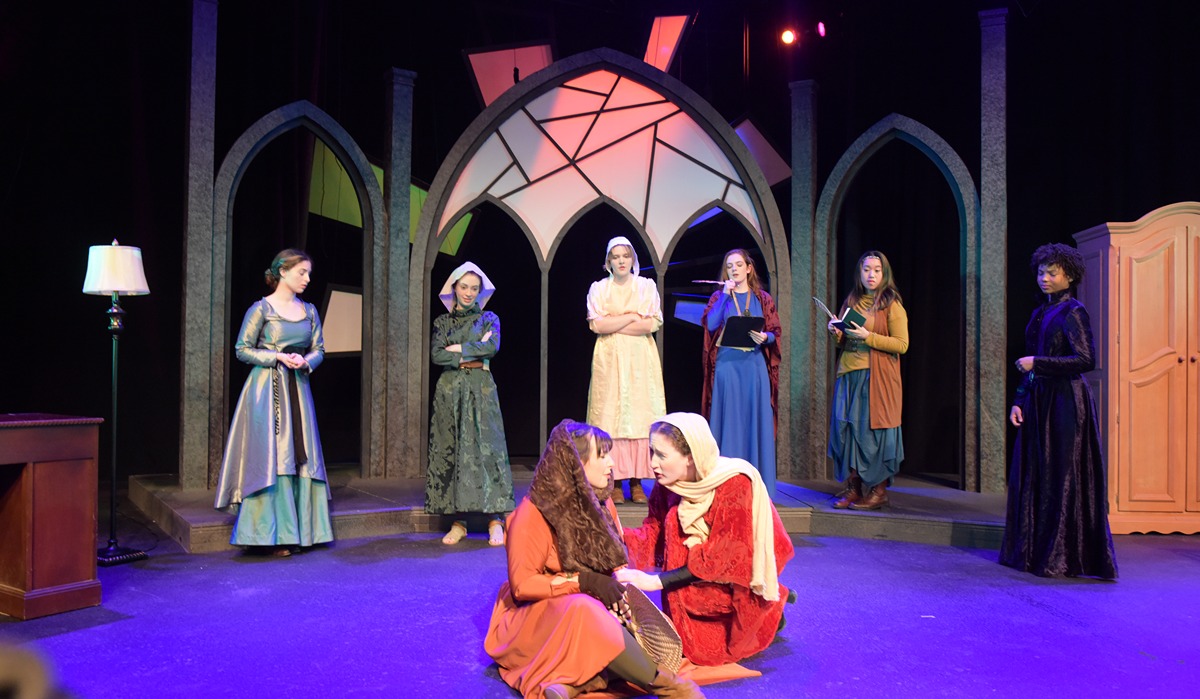The image captures a dramatic scene from a theatrical performance set against a black backdrop, framed in a wide horizontal rectangle. The stage is colored purple and features a detailed set, including a desk and a floor lamp with a white shade on the left side. Prominently, there is a striking set piece composed of three connected gray arches—two narrow at the sides framing a wider central arch with white panels at the top.

In the foreground, two central figures dressed in long dresses and head coverings crouch close together on the floor, deeply engaged with one another. One wears a red outfit with a white shawl, while the other is in a pink outfit with a brown shawl. Surrounding them are multiple women also dressed in long gowns of varying colors, such as orange, green, olive, white, blue, and brown. Some of these women are holding books and appear to be singing, collectively focusing their attention on the central pair. The intricate detail extends to accessories, with one woman on the left wearing an orange head covering and brown gloves, looking intently at her counterpart in red and white.

The set further includes a stained-glass backdrop and a series of gates and props that enhance the church-like ambiance. The cohesive yet varied costumes, the purple stage, and the thoughtful arrangement of props, like the dresser on the right, heighten the rich, immersive atmosphere of this performance.